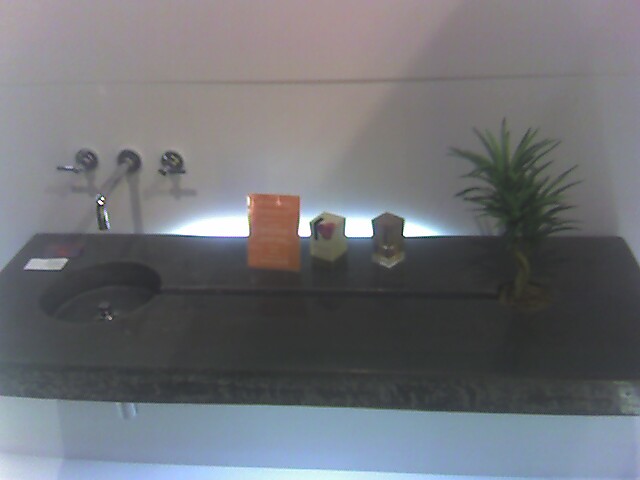The photograph captures a modern and sleek bathroom vanity counter, characterized by its dark gray color and minimalist design. The counter is essentially a floating slab without any cabinets or supports underneath, mounted elegantly against a pristine white wall. Positioned on the very left side of the counter is a round, shallow sink. The sink features a sophisticated wall-mounted faucet, which includes a silver bent metal piece and lever handles on either side for controlling the water flow.

A notable design element of this counter is a narrow groove that runs along its entire length, leading to a smaller cutout on the right, about a third the diameter of the sink. This cutout houses a potted plant, possibly a Dracaena species, recognizable by its tall, vertical, palm-like leaves.

On the back of the counter, aligned neatly behind the groove, are three distinct objects. The first is a rectangular orange plastic packaging. Next to it is a square or pillar candle, predominantly white with a black line and a red splotch on its front. The final object in this trio is a square glass vase. The counter is accentuated by a bright strip of backlighting that highlights these objects, adding a dramatic and modern touch to the overall aesthetic.